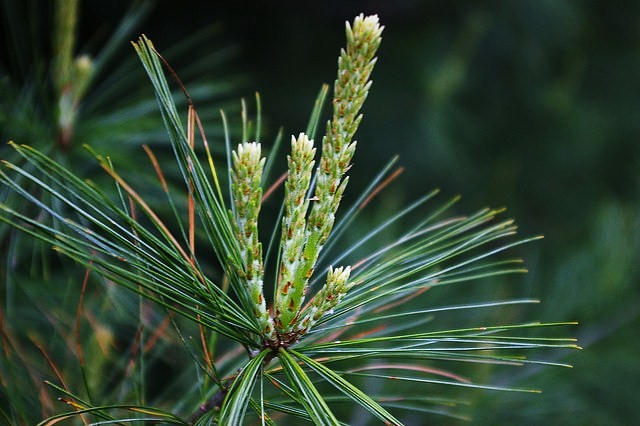This horizontal rectangular photograph captures a close-up of a plant with intricate details against a very dark, nearly black, green background. The central focus is a plant with four green, textured stalks of varying heights—one tall, two medium, and one short—surrounded at the base by an array of slender, pine needle-like leaves that spread out in a spiral pattern. The stalks, adorned with tiny green bulbs that end in white tips, resemble fresh, budding pine needles. In the blurry foreground on the right side and top right corner, additional vegetation is visible as a shadowy blob, indicating it is daytime despite the low light. A similar plant is out of focus in the top left corner, and a brown or possibly dead plant can be seen in the background. Additionally, a tree trunk on the far left adds to the composition of this detailed botanical portrait.